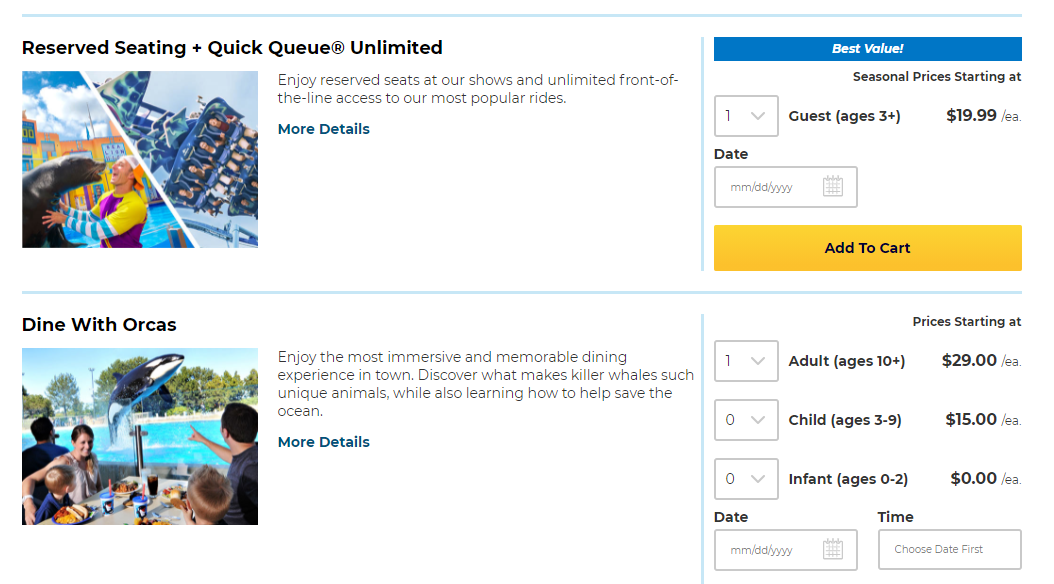This screenshot displays a webpage promoting theme park tickets with two prominent sections at the top. In the upper left corner, there is a title that reads "Reserve Seating Plus Quick Queue Unlimited." Below this title, on the left side of the page, there's a thumbnail image featuring a vibrant scene of SeaWorld: on one side, a man is interacting with a seal, and on the other, there's an exhilarating amusement park ride. The accompanying text highlights the benefits of the offer: "Enjoy reserved seats at our shows and unlimited front-of-the-line access to our most popular rides." 

Directly below this text, a "More Details" link is provided for additional information. On the right of this section, a blue banner labeled "Best Value" is prominently displayed. Underneath this banner, the text "Seasonal prices starting at" is followed by a drop-down box offering various selections. The default selection is "One guest, age 3+, $19.99 each." Beneath this drop-down box is a date selection field, and at the bottom, a conspicuous yellow "Add to Cart" button invites users to complete their purchase.